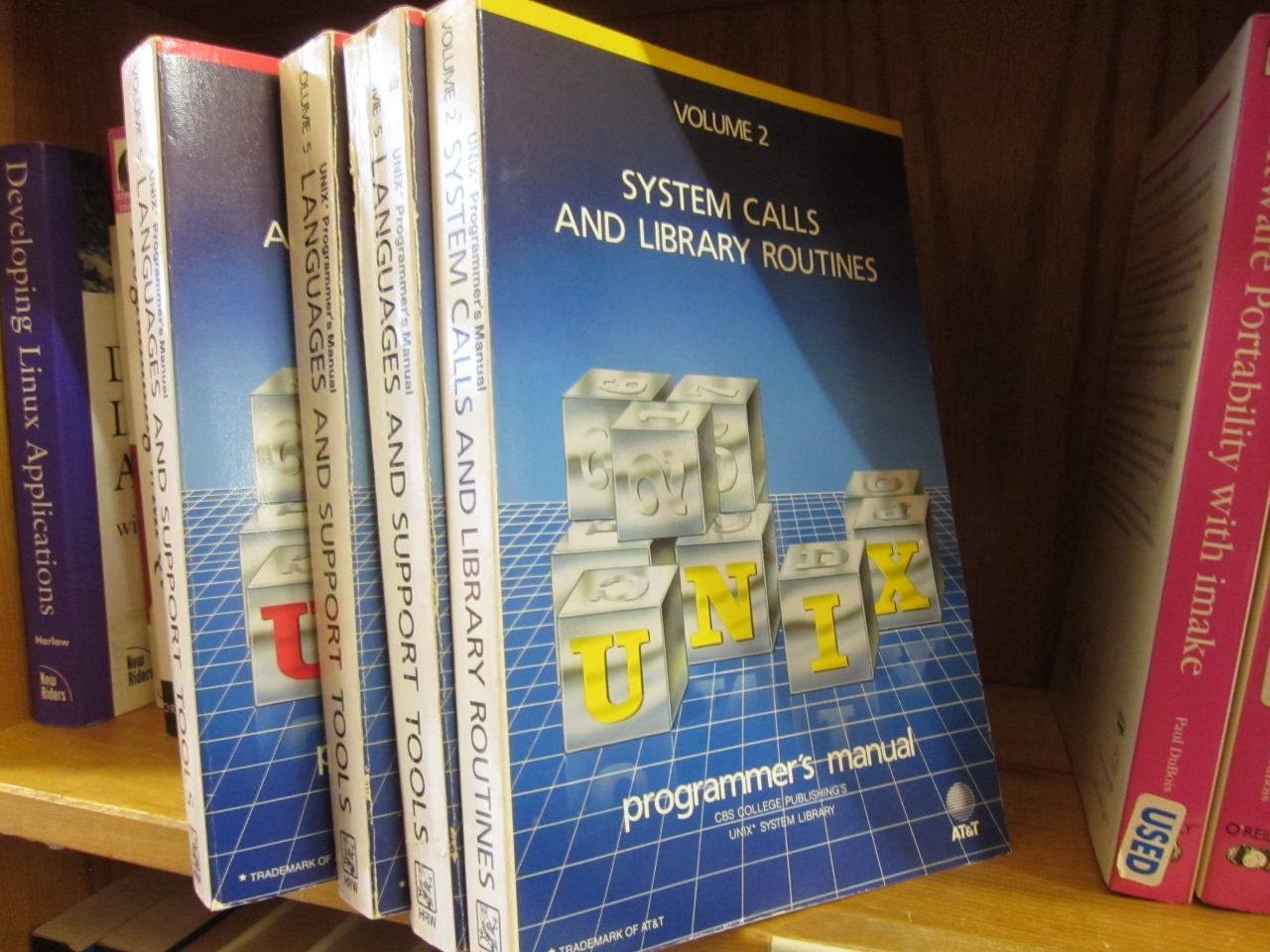This image features several computer manuals neatly arranged on a bookshelf. Dominating the foreground is a distinct book titled "Volume 2, System Calls and Library Routines," prominently marked as part of a Programmer's Manual series. The cover is adorned with metallic-like building blocks that spell out "UNIX" in yellow letters against a three-dimensional blue grid backdrop, with an overall blue shading complemented by a yellow top border. The AT&T logo is found at the bottom right corner of this book. Next to it, there is a visible title, "Developing Linux Applications," and to the right is a book with a pink cover featuring a "U" sticker. The collection suggests an array of guides and resources pertaining to languages, support tools, and Unix-based programming environments, with "System Calls and Library Routines" being a pivotal part of the series.